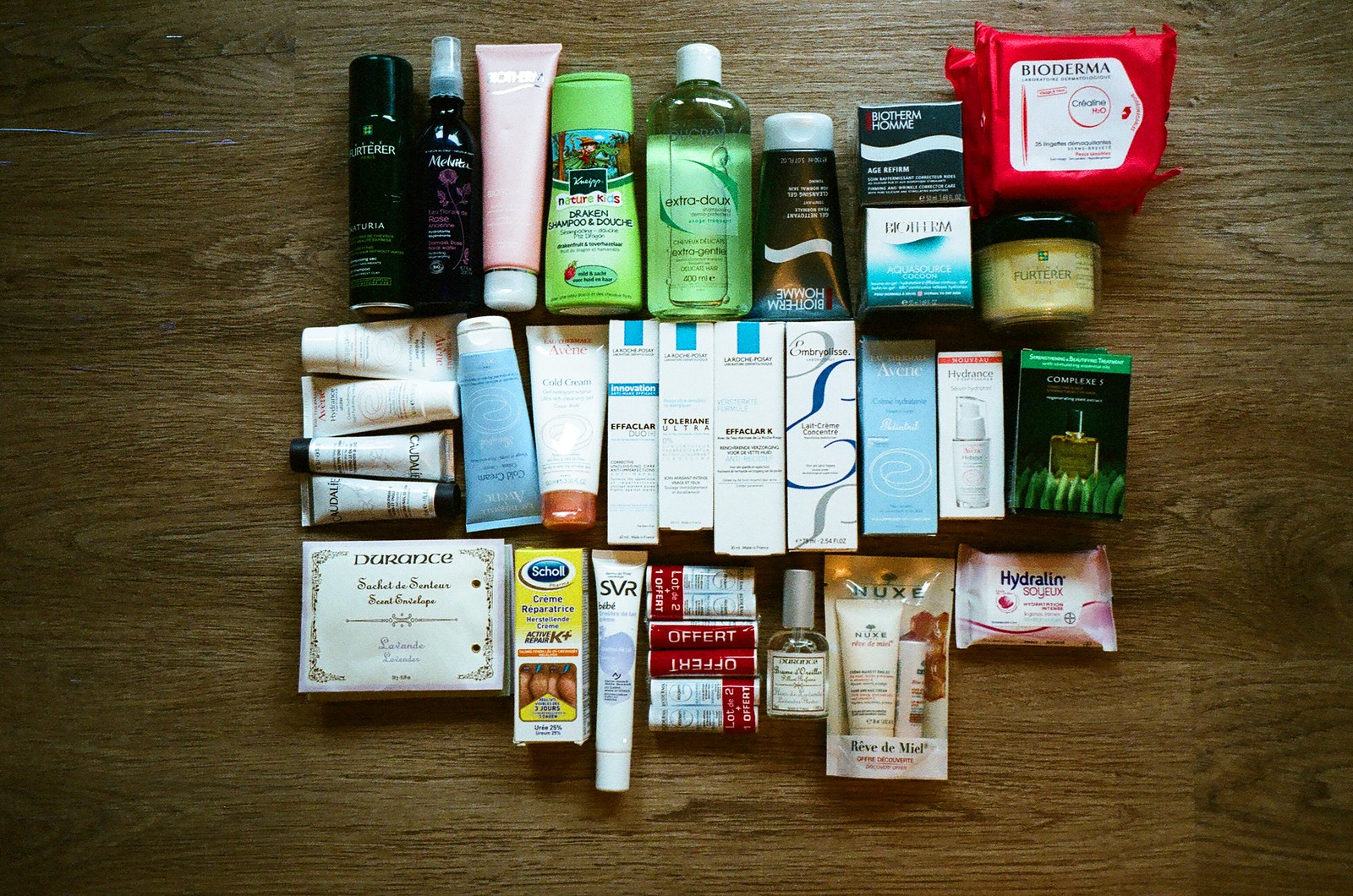The image depicts a variety of cosmetic products meticulously arranged on a brown wooden floor, showcasing the distinct planks of the flooring. From top to bottom, the layout is as follows:

- Top row (from left to right):
  - A black aerosol can with white and green lettering, likely indicating a can of hairspray.
  - A dark spray bottle, labeled possibly with "Marrakesh," suggesting it is a hair spray.
  - A pink tube with a white cap at the bottom.
  - A green bottle with a flip-top lid and some writing on it.
  - Another green bottle, containing liquid, with a green screw-cap flip-top.
  - A brown tube positioned upside down with a white flip cap and white writing.
  - Two square boxes stacked on each other— the top box is black with a white squiggle and writing, and the bottom one is white with blue accents.
  - A white-labeled Bioderma product with black writing and red packaging, possibly containing wipes.
  - A yellow item, which could be a tube or box, with a black screw cap.
  
- Second row (from left to right):
  - Four white tubes.
  - A blue tube with a white cap.
  - A white tube with a brown cap, oriented inversely.
  - Three boxes, predominantly white at the bottom with blue tops—likely La Roche-Posay products.
  - A white box with blue writing.
  - A blue box.
  - Another white box.
  - A smaller black box with green writing.

- Bottom row (from left to right):
  - A white rectangular package.
  - A Dr. Scholl's product, probably for foot care.
  - A white tube.
  - Six additional white tubes.
  - A clear nail polish bottle.
  - A package containing lotion and chapstick.
  - A pink package labeled "Hydrolyn."

This organized display highlights an array of skincare, haircare, and personal hygiene items, including various sprays, tubes, bottles, and boxed products, showcasing a thorough collection of beauty and healthcare essentials.